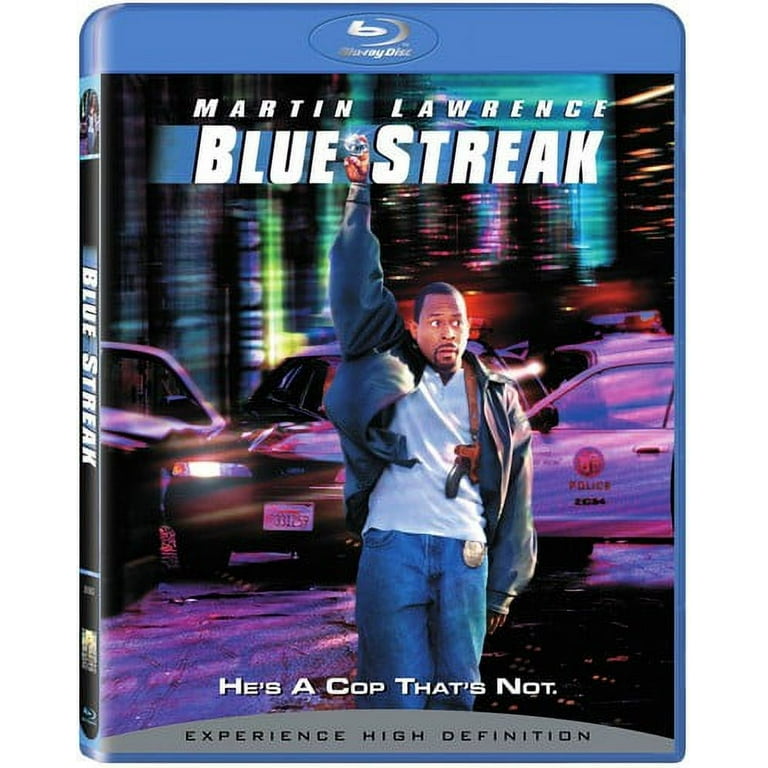This image is a portrait-oriented photograph of a Blu-ray disc cover for the movie "Blue Streak," featuring Martin Lawrence. The Blu-ray case has a sky-blue background. At the top, the Blu-ray Disc logo is visible, followed by the movie's label, which features "Martin Lawrence" in white letters. Beneath his name, "Blue Streak" is prominently displayed in large white letters with a hint of blue background. The tagline, "He's a cop that's not," appears below the title. Martin Lawrence is depicted standing on the cover, wearing a gray jacket, a white shirt, and jeans, with a gun holstered around his chest and a police badge hanging from his jeans. He is holding one hand in a humorous gesture between the words "blue" and "streak," looking off to the right. Behind him, you can see three cop cars and a blur of swirling city lights in black, purple, green, and blue. At the bottom of the cover, in a gray arc, the text reads "Experience high definition" in black. The spine of the Blu-ray case also displays the title "Blue Streak" in white letters.